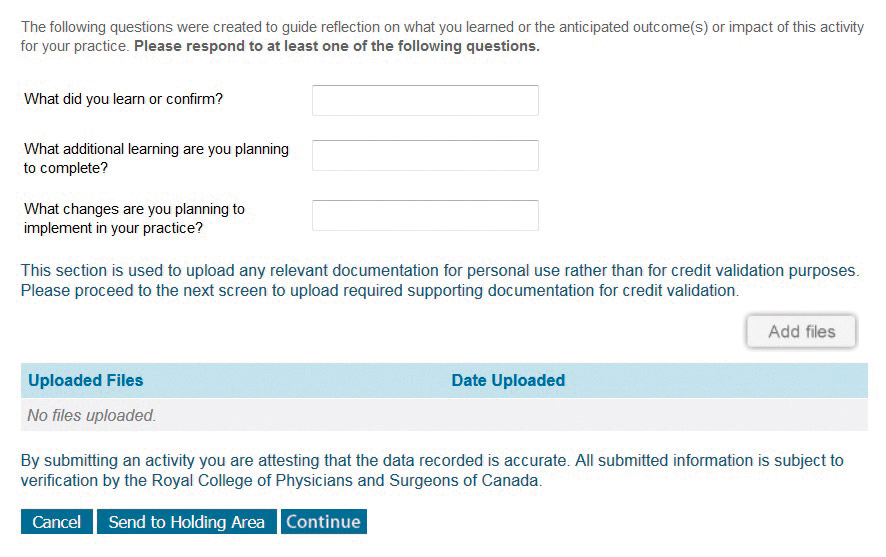Caption: This is a detailed view of the recap area provided at the end of an online lesson, quiz, or test. The header at the top states, "The following questions were created to guide reflection on what you learned or the anticipated outcomes or the impact of this activity for your practice. Please respond to at least one of the following questions." Below, it lists three reflective questions with blank input fields for responses:
1. What did you learn to confirm? 
2. What additional learning are you planning to complete? 
3. What changes are you planning to implement in your practice?

Below these questions, a section marked in blue text indicates that this area is used to upload relevant documentation for personal use rather than for credit validation purposes. To upload the required supporting documentation for credit validation, users must proceed to the next screen.

A button in the lower right corner, labeled "Add Files," allows the user to upload files. Directly beneath this upload button, there is a light blue bar displaying the status of any uploaded files, which currently shows "No files uploaded" in gray text. 

Further down, a statement reads, "By submitting an activity you are attesting that the data recorded is accurate. All submitted information is subject to verification by the Royal College of Physicians and Surgeons of Canada." 

In the lower left corner, there are three dark blue buttons with large white text offering the following options: "Cancel," "Send to Holding Area," and "Continue." The rest of the screen is blank with ample spacing between each of these sections, providing a clean and organized layout.